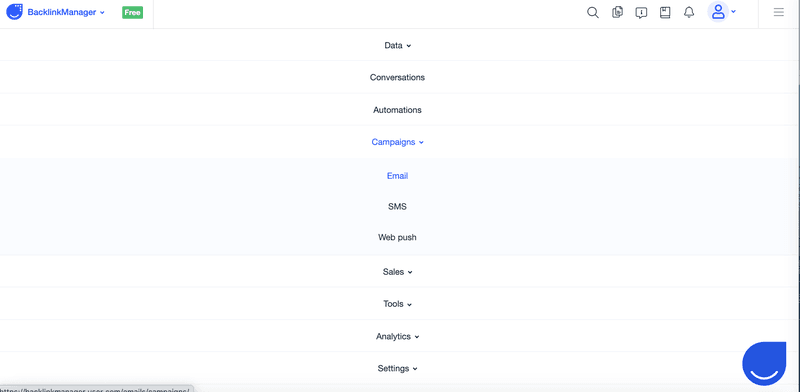The image features a blue circular icon wearing a small triangular cap, resembling a face with a white smile at the bottom. Adjacent to this icon are some blue text and a green rectangle containing white text, both of which are unreadable. To the right, there are several symbols: a magnifying glass, an unidentifiable icon, a speech bubble-like figure with contents, two overlapping squares, a bell, a blue circle with a person icon and a dot, and three stacked gray lines. Below this toolbar, the center column lists the following words vertically: "Data," "Conversations," "Automations," and, in blue, "Campaigns" accompanied by a downward arrow. Further down, the following items are listed in blue with accompanying downward arrows: "Email," "SMB," "Web Push," "Sales," "Tools," "Analytics," and "Settings." The left side of the image contains a gray section, while another circular icon with a triangular cap and white smile appears on the right.